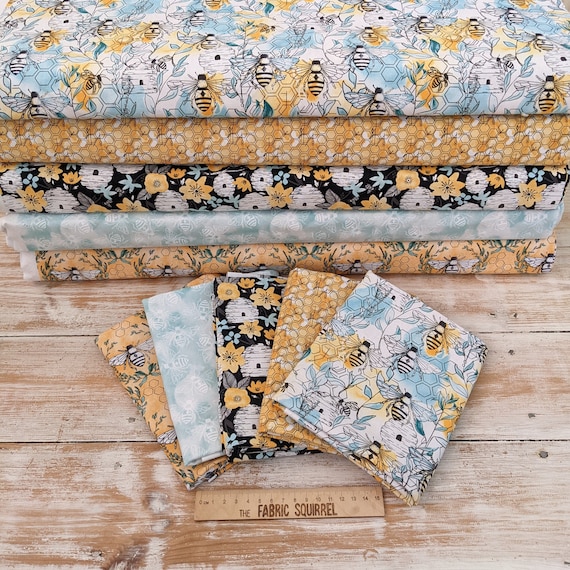The image features a promotional display for "The Fabric Squirrel," showcasing five bolts of fabric, each with unique yet cohesive designs centered around a honeybee and flower theme. The fabrics are neatly stacked in the background, arranged from top to bottom with patterns including bumblebees against a blue and white honeycomb background, a gold, yellow, and white honeycomb, and black, yellow, and white flowers. Additional designs include a blue-themed fabric and another bee pattern. These bolts are placed on a wooden floor or table. In the foreground, smaller squares of each fabric pattern are arranged in an overlapping fan formation, accompanied by a one-foot ruler. The promotional text "The Fabric Squirrel" is prominently displayed, indicating the name of the business or brand.